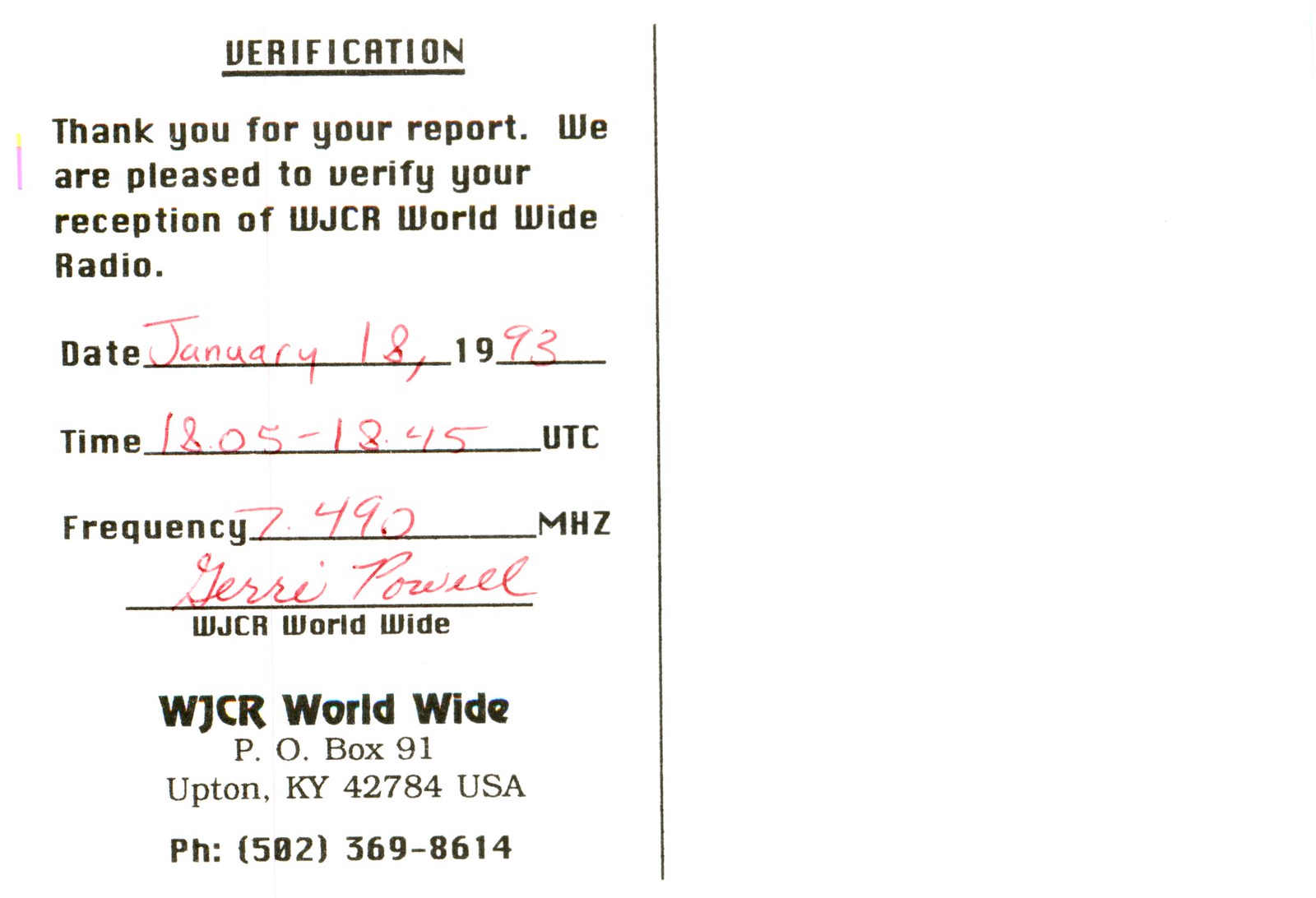The image displays a verification form titled "VERIFICATION" at the top, underlined for emphasis. Below it is a message that reads, "Thank you for your report. We are pleased to verify your reception of WJCR Worldwide Radio." Following this, there are handwritten details in red pen, including the date "January 18th, 1993," the time span "1805 to 1845 UTC," and the frequency "7.490 MHz." The form is signed by Jerry Powell, representing WJCR Worldwide. At the bottom of the form, the contact information for WJCR Worldwide is listed: "WJCR Worldwide, PO Box 91, Upton, Kentucky, 42784 USA," along with the phone number "502-369-8614." The layout and elements of the form resemble the back of a postcard, with a vertical rule typically used to separate the address from the message.